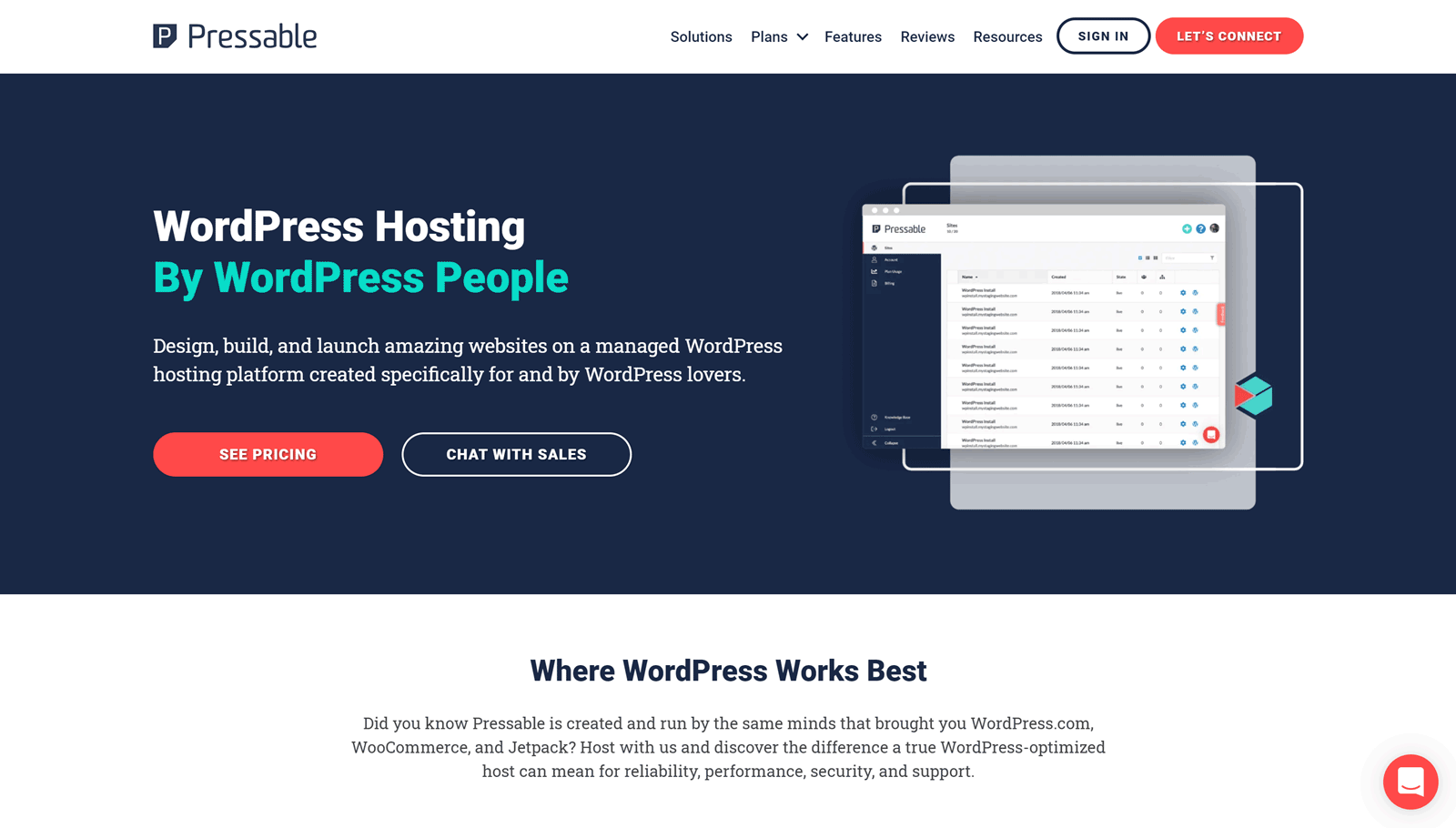This advertisement for Pressable, a WordPress hosting service, is featured prominently on our website. 

In the upper left corner, a logo consists of a white "P" inside a navy blue rectangle with a folded bottom right corner, accompanied by the name "Pressable." A navigation menu includes the following options: "Menus," "Solutions," "Plans" with a drop-down arrow, "Features," "Reviews," and "Resources." To the right of the menu, there is a navy oval "Sign In" button with the text in navy blue, and a red oval "Let's Connect" button with white text.

Below this, a large navy blue rectangle serves as the main advertisement area. It features "WordPress Hosting" in white text and "By WordPress People" in aqua blue text. A tagline in white reads, "Design, Build, and Launch Amazing Websites on a Managed WordPress Hosting Platform Created Specifically for and by WordPress Lovers." Two buttons are located at the bottom of this section: a red "See Pricing" button with white text, and a blue "Chat with Sales" button with white text and a white border.

On the right-hand side of the advertisement, there is another "Pressable" logo and a depiction of the UI for working with WordPress, although the interface details are somewhat difficult to discern. 

Below the main rectangular section, against a white background, blue text states "Where WordPress Works Best," followed by black text noting, "Did You Know Pressable is created and run by the same minds that brought you WordPress.com, WooCommerce, and Jetpack? Host with us and discover the difference a true WordPress-optimized host can mean for reliability, performance, security, and support."

Additionally, on the right-hand side, an orange circle containing a speech bubble with an orange smiley face is visible, adding a touch of friendly character to the advertisement.